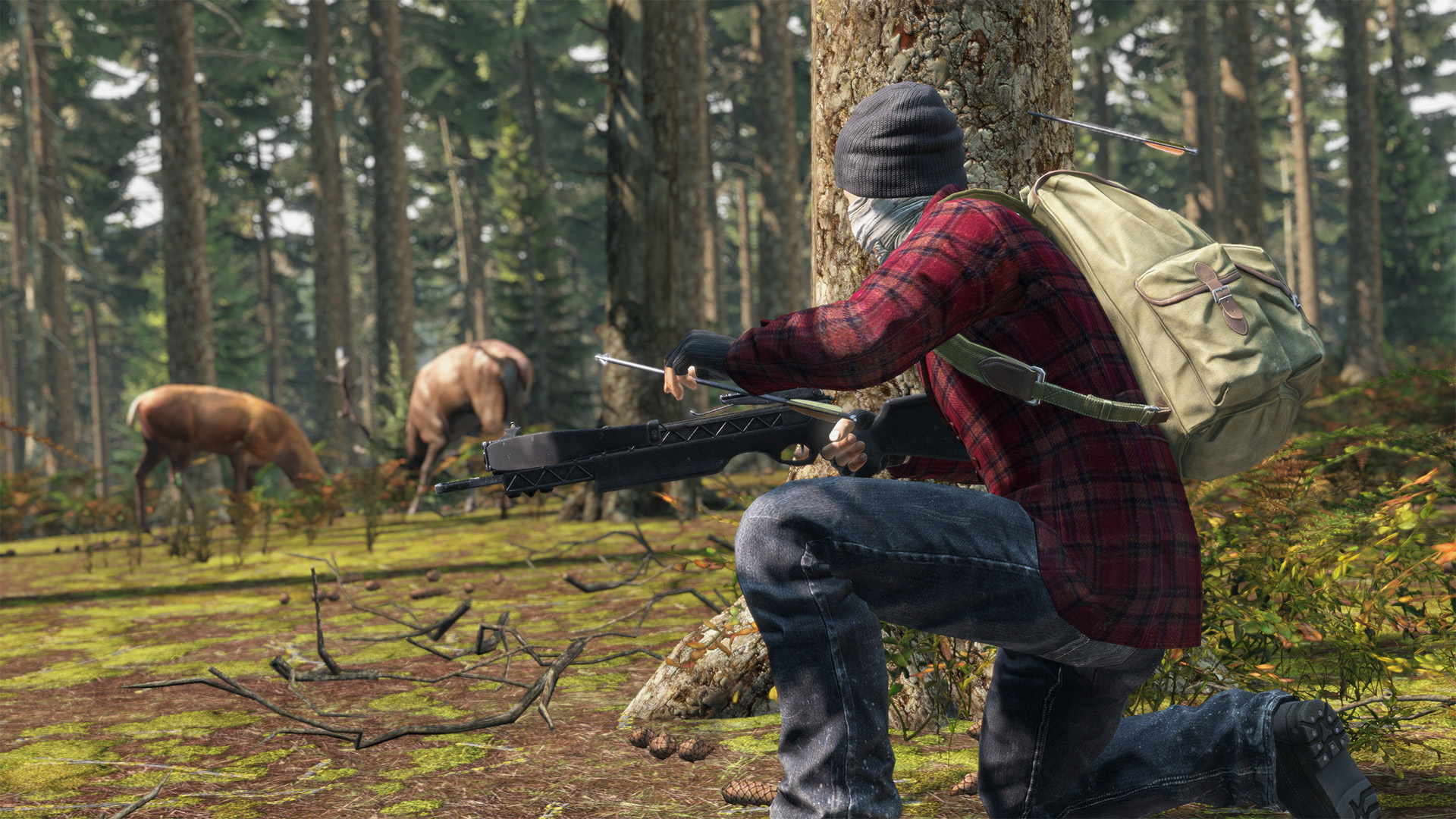In this detailed screenshot from what appears to be a hunting video game reminiscent of DayZ or Days Gone, we observe a character partially concealed behind a large tree in the center, which has an arrow embedded slightly off-center to the right. The character, depicted from a side angle, is in the midst of loading an automatic hunting bow. They are attired in a red and blue plaid shirt, blue jeans, and black boots, with a tan backpack strapped on their back. The character also sports a black beanie, with strands of white or blue hair visible beneath it. Additionally, they wear a face mask and have a walkie-talkie attached. In the background, the forested terrain reveals two deer grazing to the left of the character; one is a male with prominent antlers, and the other appears to be a female. This scene encapsulates the quintessential elements of a survival or hunting-themed game, blending suspense with the intricacies of tracking wildlife.